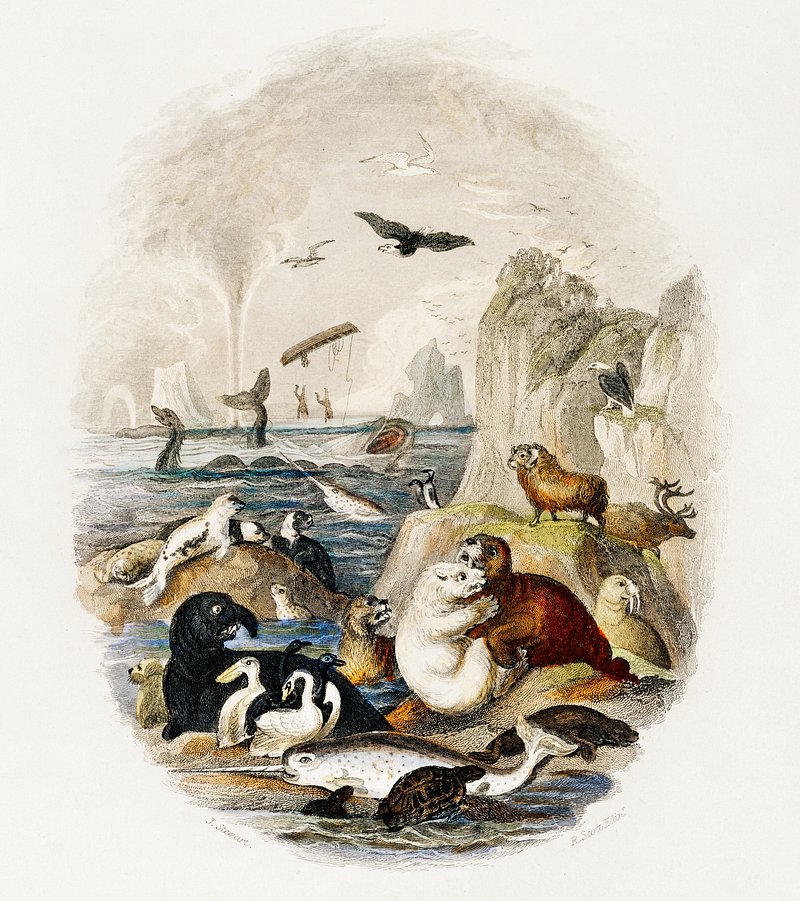This highly detailed and vivid color illustration on white paper features a bustling rocky shoreline scene viewed through a circular window format situated in the middle of the image. The foreground is alive with activity as brown and white seals engage in a playful wrestle while a swordfish lies on the bank beside them. Numerous seabirds are either perched on stones or soaring above the scene, including an eagle. Walruses, including a prominent black one, and a large turtle emerge from the water, adding to the rich diversity of sea life on display. In the ocean, a narwhal is seen facing left, almost looking at the viewer with its distinctive horn protruding from the water. Behind the narwhal, a creature resembling a sea serpent or the Loch Ness monster glides through the water. Nearby, a dramatic scene unfolds as a whale appears to capsize a boat, sending two men plunging into the sea. The backdrop reveals a picturesque rocky outcropping with cliffs to the right, while on the left, a grand water spout ascends towards the cloudy, overcast sky. The artist, J. Stewart, has signed their name at the bottom left of this intricate and dynamic illustration.